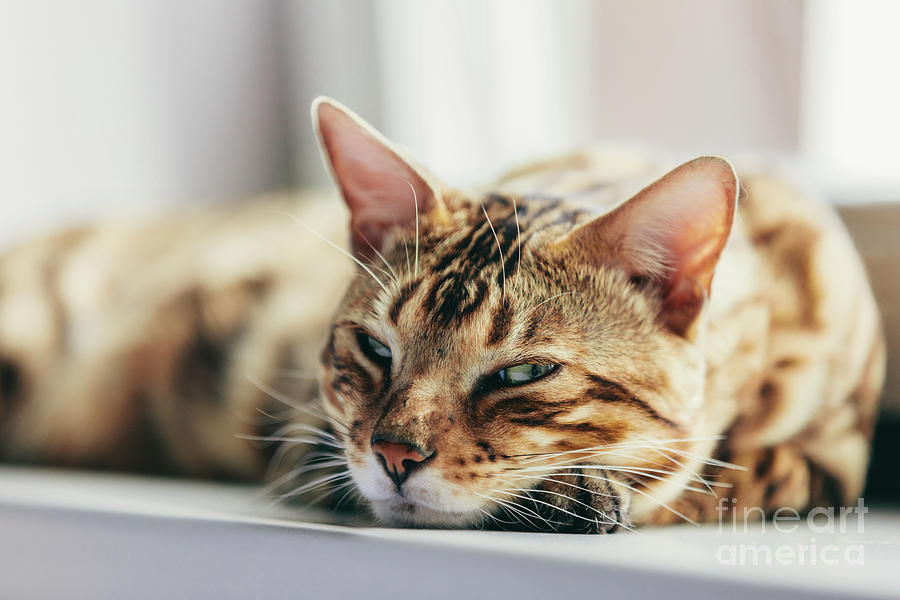This image portrays a serene moment of a tan and black striped cat resting on a white ledge, possibly the edge of a chair or a wall-mounted bench. The soft, natural light filters through two windows in the background, gently illuminating the scene. The cat's partially closed eyes suggest it is on the verge of drifting into a nap, its little pink nose adding a touch of delicate charm. The cat's head is laid down gently on its paws, with the front part of its face in sharp focus, capturing fine details of its fur and markings. The rest of the cat's body and the background are artistically blurred, emphasizing the tranquility of this peaceful moment.